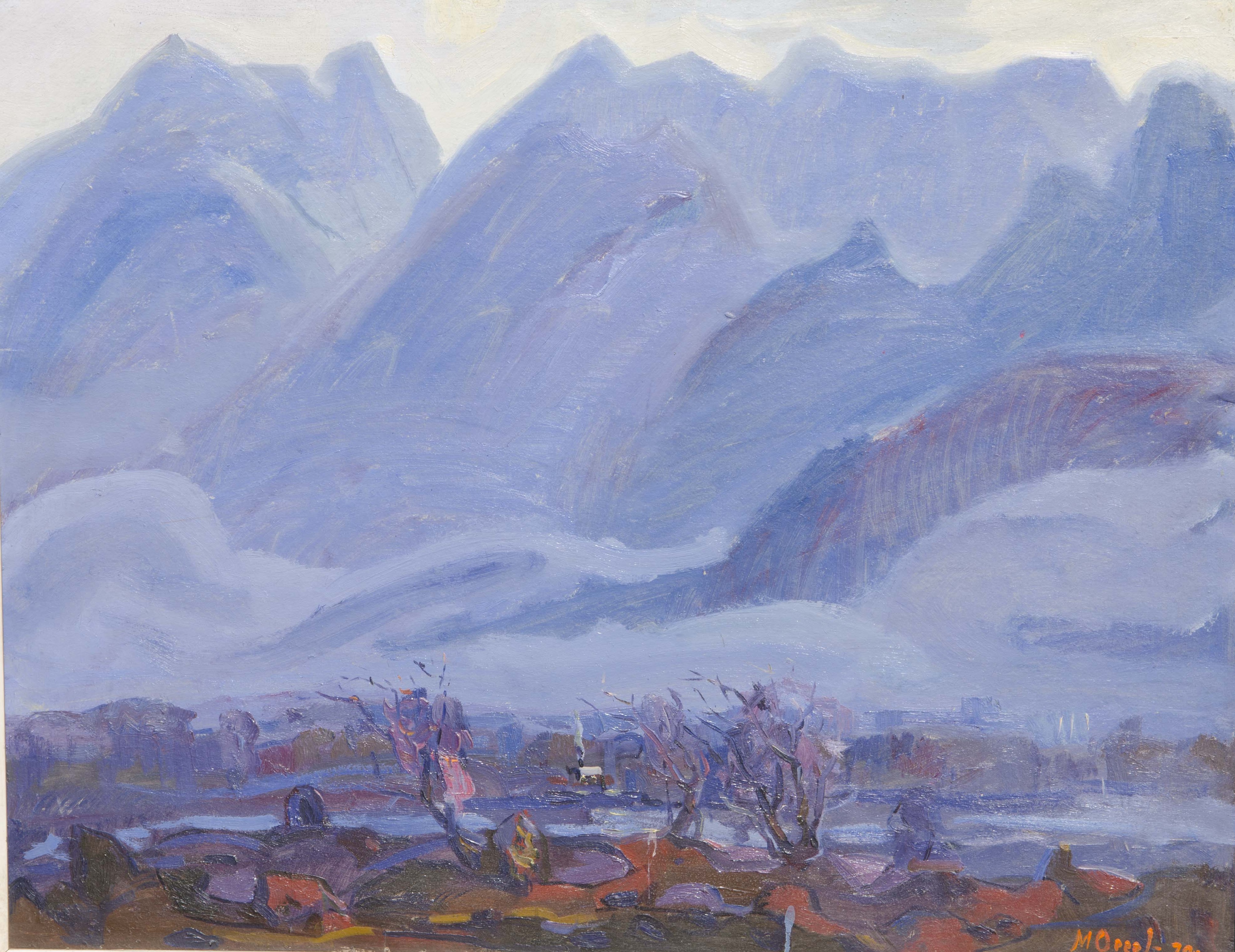A large square painting without a border depicts a dramatic landscape scene. The composition starts at the top with a white and gray sky filled with clouds, immediately giving way to imposing blue-gray mountains. The mountains, rendered in varying shades of gray and blue, dominate much of the scene, their swirling lines creating a sense of immense height and ruggedness. The mountain range consists of shorter peaks in the foreground and taller peaks extending into the background, suggesting depth and scale. 

Below these mountains is a cliffside characterized by brown and gray hues, which seamlessly transitions into a turbulent body of water marked by large, whitish-gray and blue waves. In the mid-ground, hovering just above a barren, desert-like earth, the abstract outlines of buildings in shades of brown, red, gray, and black create the silhouette of a deserted town, their rectangular shapes hinting at windows and deserted facades. 

The foreground is a stark contrast, featuring a scraggly, leafless landscape with clay-colored dirt, various shades of brown indicating rocks and barren ground, and a few bare branches and possibly small trees. In the lower right-hand corner, partially obscured letters "M-O" suggest an artist’s signature. The entire painting has a chalky texture, adding to its abstract and desolated atmosphere.